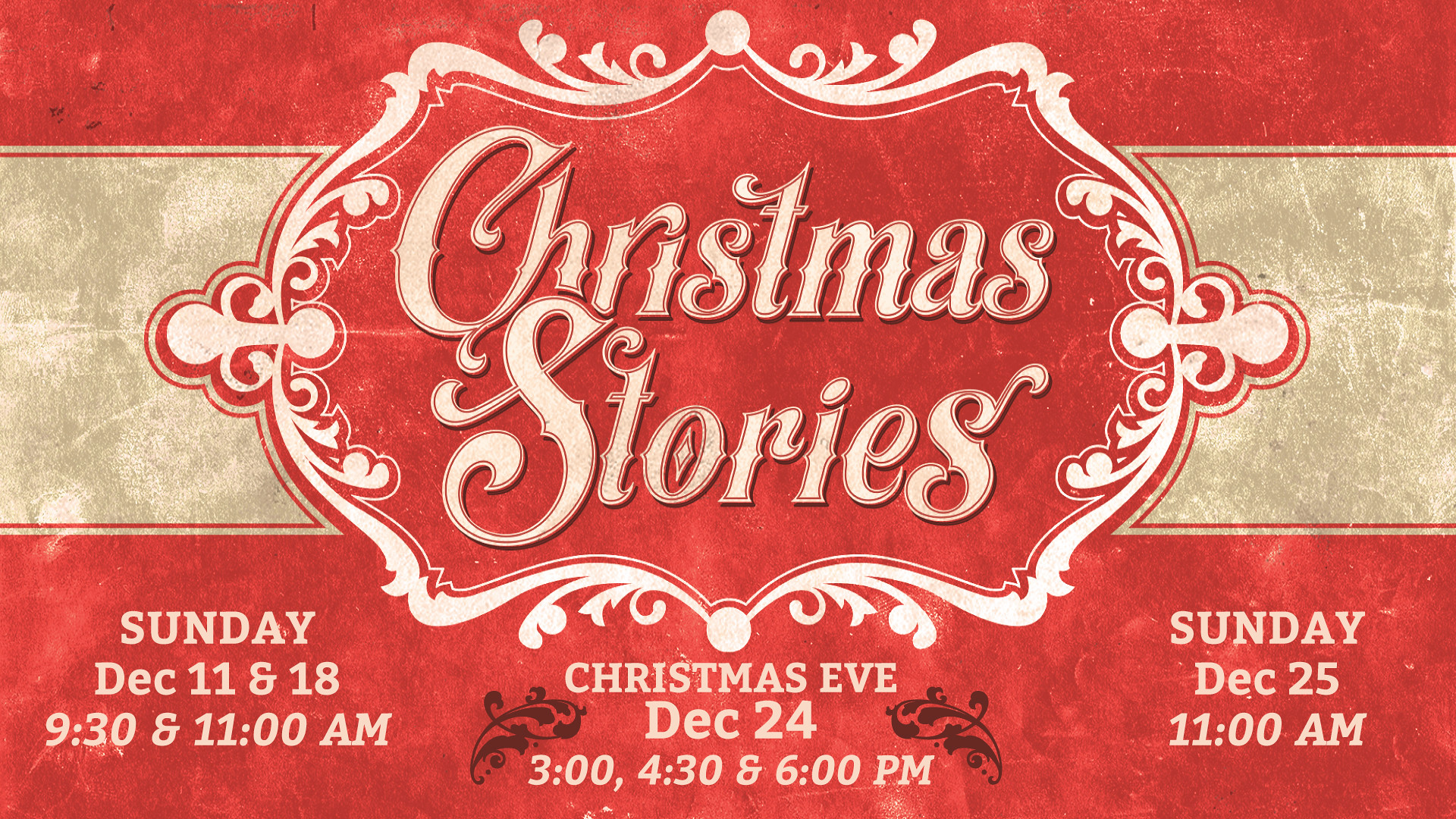This advertisement features a festive holiday design with a red and beige color scheme. At the top and bottom are horizontal red stripes, creating a flag-like appearance. The central beige stripe, which looks aged and leathery, houses an ornate white frame. Inside this frame, in an elegant and elaborate italicized font, the text "Christmas Stories" is prominently displayed. Below this central text, the event details are listed:

- **Sunday, December 11th and 18th**: 9:30 AM and 11:00 AM
- **Christmas Eve (December 24th)**: 3:00 PM, 4:30 PM, and 6:00 PM
- **Sunday, December 25th**: 11:00 AM

These dates and times are printed clearly within the red bands at the bottom, each set of times bracketed by ornate designs. The overall aesthetic conveys a vintage holiday charm, making it an inviting announcement for seasonal festivities.